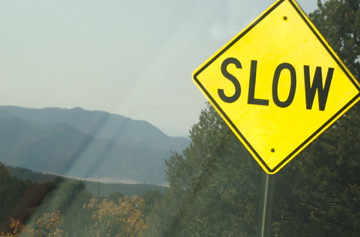This color photograph captures a scenic mountain landscape dominated by a yellow diamond-shaped street sign that reads "SLOW" in bold black letters, bordered by a thin black line. The sign is mounted on a standard metal pole. The background reveals a daylight scene featuring an array of evergreen trees interspersed with some displaying fall colors of red, gold, and green. The distant mountain ranges ascend high into the sky, which appears overcast and gray, fading paler near the horizon where it meets the mountains. Sunbeams diagonally cut across the scene from the top edge, slightly right of the center, to the bottom left corner, imparting a glare that suggests the photo might have been taken through a window, potentially from inside a car. The overall image exudes a serene yet cautionary atmosphere with no people, animals, or buildings present.